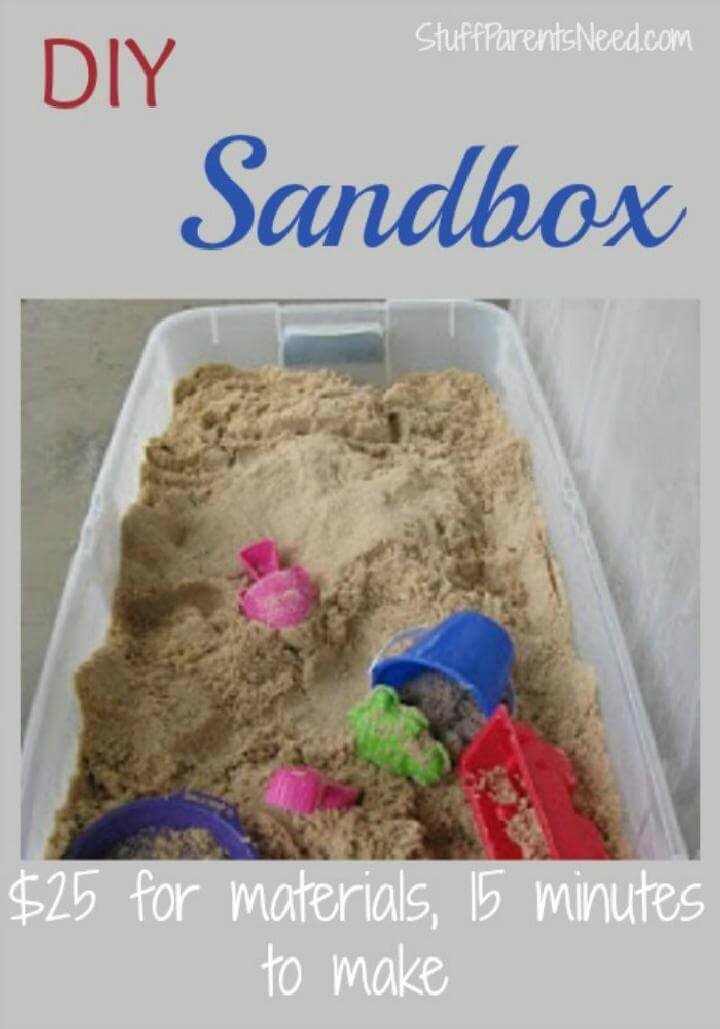The image appears to be an informational poster or the front cover of a magazine, promoting a DIY sandbox project. The tall, rectangular layout resembles a book cover, with a gray background at the top and bottom. At the top, bold red letters spell "DIY," followed by "Sandbox" in large blue font. In the top right corner, the website URL "StuffParentsNeed.com" is displayed in white text. Below the title is a photo of the DIY sandbox—a large, clear plastic storage tote filled with beige sand. The sandbox contains a variety of colorful plastic toys, including a pink shovel, a blue bucket, a green turtle mold, and other small molds and shovels in red and blue. The bottom of the poster notes that the materials cost $25 and the project takes only 15 minutes to complete, making it a quick and affordable activity for kids.